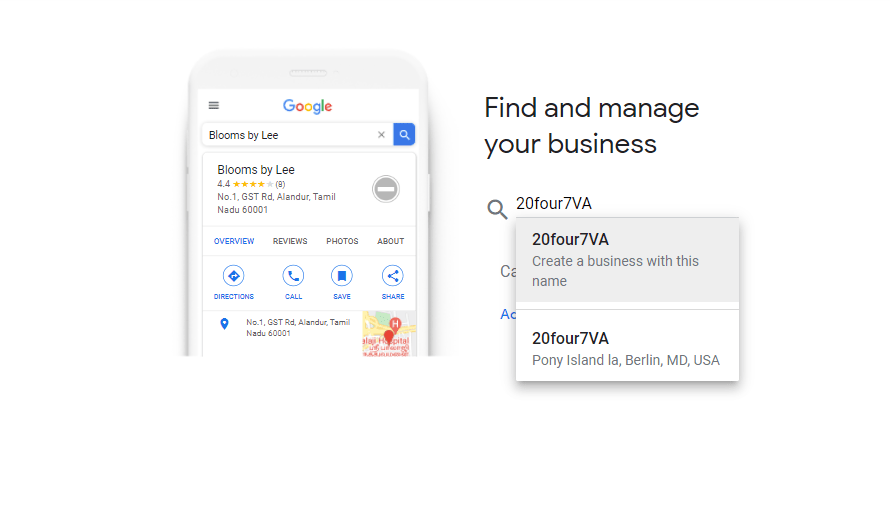This image appears to be a promotional screen capture, likely for an advertisement prototype, showcasing a user interface designed for a business. 

The ad is set against a clean white background and features an older model cell phone. The cell phone's screen prominently displays the Google search interface. On the left side of the screen, there are three black lines, typically representing a menu icon, followed by the multicolored Google logo with a blue "G," red "O," yellow "O," blue "G," green "L," and red "E." Below the logo, a white search box is visible with the text "Blooms by Lee." Adjacent to the search box is a gray 'X' icon and a blue box containing a white magnifying glass, indicative of the search function.

The page showcased on the screen provides business details for "Blooms by Lee," which has a 4.4-star rating based on 9 reviews. The listed address is "No. 1 GST Road, Aldor, Tamil Nadu, 60001." Beneath the business name and its rating is a gray circle with a white minus sign, likely used to collapse or reduce details. The interface displays tabs for "Overview," "Reviews," "Photos," and "About," with the "Overview" section highlighted in blue to signify its active status.

Further down the screen, action buttons for "Directions," "Call," "Save," and "Share" are displayed, each paired with respective icons. The business address is reiterated at the bottom, accompanied by a blue location pin icon. A small map segment is visible in the corner, showing areas colored in yellow, green, and red.

On the right side of the image, the ad text reads "Find and Manage Your Business" in bold black letters, accompanied by a magnifying glass icon. Below, text in black reads "247VA," followed by a small white box. The box, containing options for business creation, displays “247VA, create a business with this name” and "247VA, Pony Island, LA, Berlin, Maryland, USA."

This detailed presentation highlights the process for managing and finding businesses on a Google-like search platform, offering a glimpse into user interactions with business listings and creation.